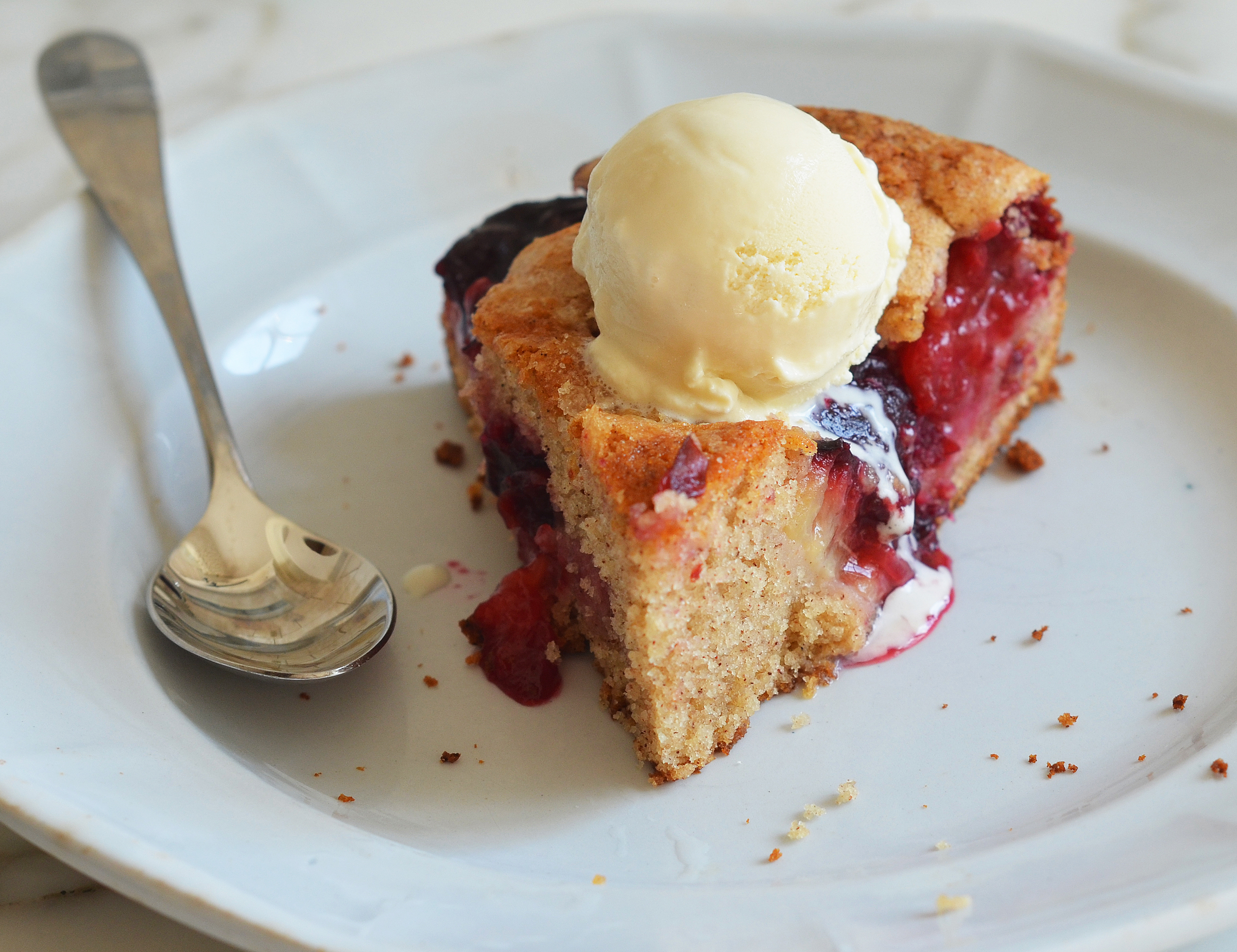This detailed close-up photograph captures a delectable dessert presented in a white porcelain shallow bowl. The dessert is a large, pie-shaped wedge that suggests more of a cobbler than a traditional pie, as it lacks a visible crust but features ample golden, puffy dough. The filling comprises a medley of dark reddish-bluish berries, possibly cherries or mixed berries, giving it a rich, juicy appearance. 

A generous scoop of slightly butter-hued French vanilla ice cream crowns the dessert, beginning to melt and cascade over the sides. The ice cream forms a flawless, circular dollop that enhances the visual appeal of the dish. On the left side of the bowl, a spoon rests with its bowl facing the camera and handle extending toward the upper left corner. Although some crumbs are scattered around indicating the texture of the dessert, the spoon remains untouched, ensuring the anticipation of tasting this inviting treat.

The bowl sits on a white plate, itself placed on a smooth white marble countertop with subtle gray veining, adding a touch of elegance to the setting. Crumbs surround the dessert, evidence of its crumbly, tender composition, making this a picture-perfect indulgence waiting to be enjoyed.